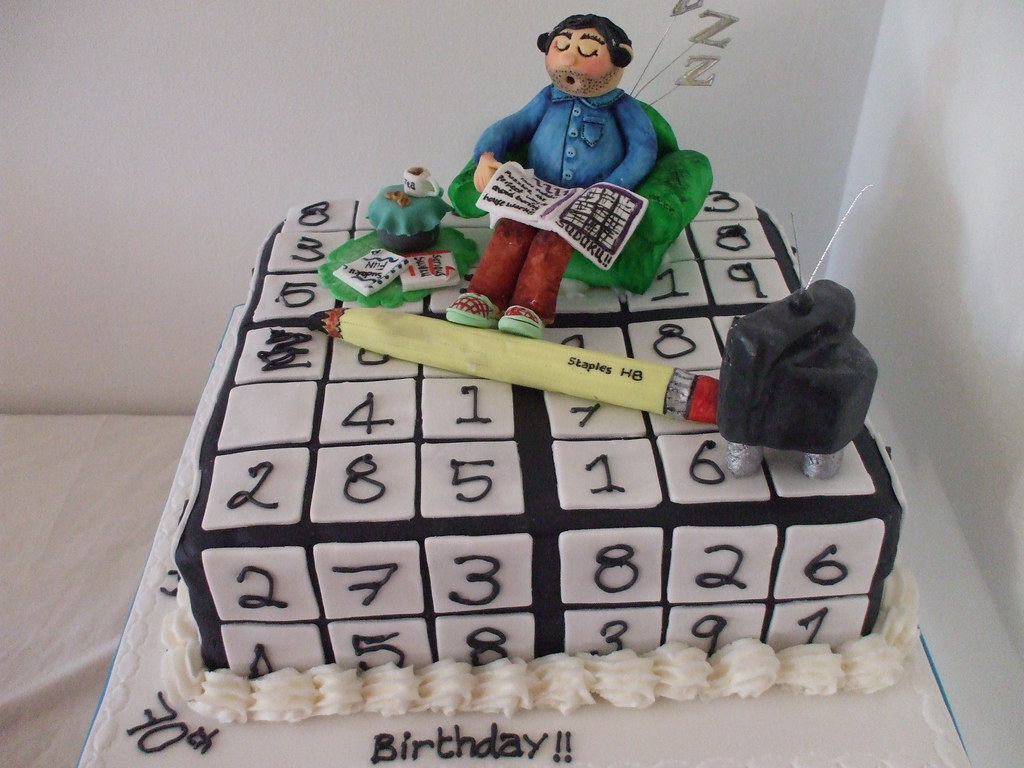This is an image of a unique and creatively decorated 70th birthday cake. The cake, placed inside a white paper box, is square-shaped with white frosting and black borders. The surface design mimics a Sudoku puzzle with various numbers such as 2, 7, 3, 8, 2, 6, 4, 5, 8, 3, 9, and 1 arranged across the squares. Resting on top of the cake is an intricate, playful scene featuring a toy figure of a man in a blue shirt and red pants, sitting on a green chair with his eyes closed and marked with 'Z's to indicate he is sleeping. The man, who has black hair, is holding a yellow Staples HB pencil under his feet and has a newspaper or magazine to his left with additional books and a coffee mug on a table nearby. A small TV set is also part of the scene, enhancing the whimsical detail. The cake features a frilly cream border around its base and is labeled "70th birthday" at the bottom in white icing. The overall effect is a combination of a Sudoku puzzle and a cozy, humorous depiction of someone asleep amidst their hobby.